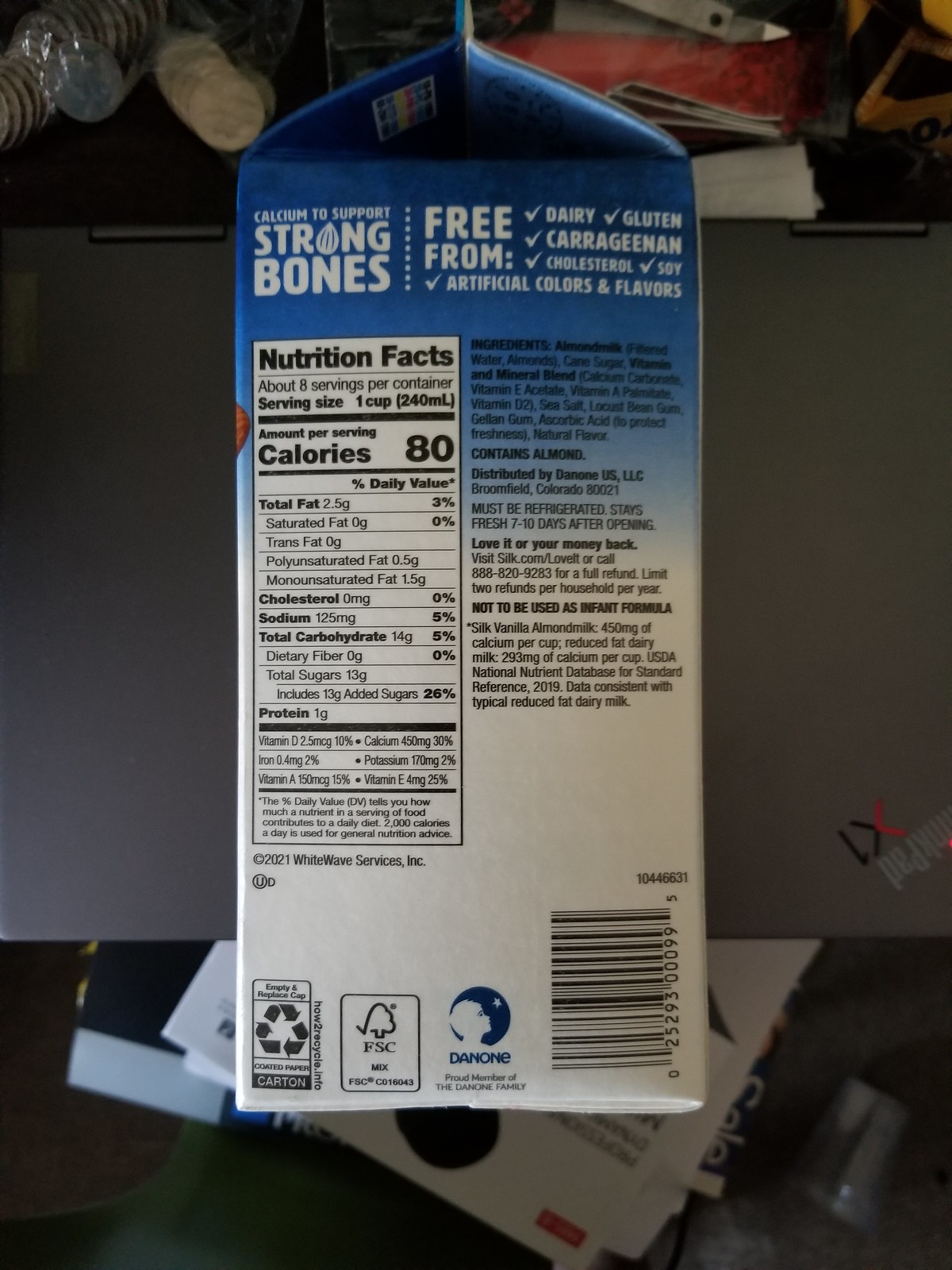In this image, we see the side of an almond milk carton prominently displaying its Nutrition Facts. The carton, labeled with "calcium to support strong bones," declares that the almond milk contains 80 calories per serving. It is positioned on a ThinkPad laptop, viewed from above, and distributed by Danone, as indicated on the carton. In the upper left corner of the frame, an open bag of Ritz crackers is partially visible, adding context to the setting. The scene combines the detailed presentation of the almond milk's nutritional benefits with everyday elements like a laptop and snacks, creating a relatable and everyday atmosphere.